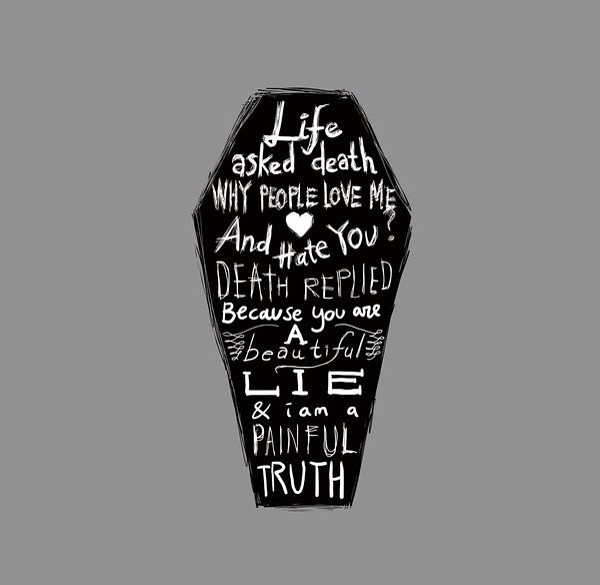The image features a drawing of a coffin-shaped sign with a unique design that is reminiscent of a casket or a mummy case. The sign is predominantly black with flared sides and a square top and bottom. Displayed on the sign is a poignant dialogue written in white handwritten text. At the top, it begins with "Life asked Death," followed by the question, "Why do people love me and hate you?" A small white heart against the black background separates "love me" and "hate you," with a question mark following "hate you." The response from Death reads, "Because you are a beautiful lie and I am a painful truth," with the word "beautiful" elegantly written in cursive with decorative loops extending from the letter 'A'. The entire text, though handwritten and not typeset, captures a profound exchange emphasizing the contrasting perceptions of life and death.